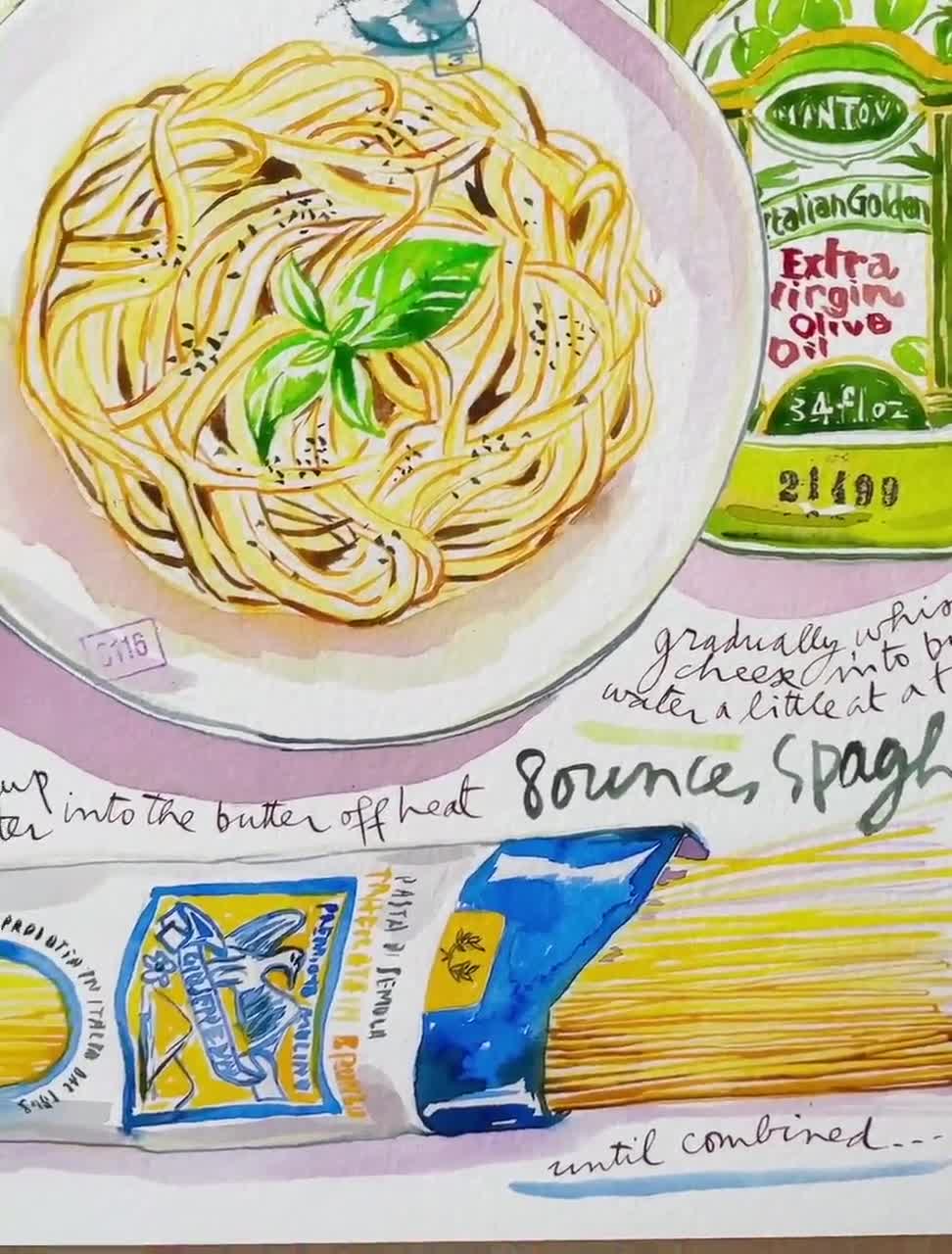The image is a detailed watercolor drawing of a culinary scene depicting a plate of spaghetti, or possibly long curved pasta, with a green leaf garnish on top, all set on a white and pink plate. In the upper right corner, there is a green bottle labeled "Italian Golden Extra Virgin Olive Oil" in red text, with an unclear volume measurement, possibly "3.4" or "34" fluid ounces. Nearby, there's a package with yellow pasta, and an unclear brand name, possibly "Mantov." Below this, there is text that appears to be partial cooking instructions, stating: "Gradually whisk cheese into boiling water a little at a time, then into the butter off heat," and "stir until combined." The bottom of the image has an unclear number, "21499," and a depiction of uncooked spaghetti, suggesting a step in the recipe.